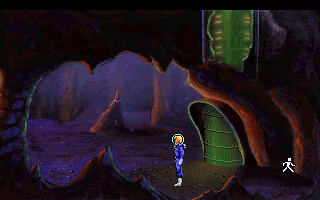The image is a screenshot from a retro-style video game, reminiscent of classic adventure or text-based games, but with visually animated characters. The scene is set in a cave with brown walls and a darker, almost black background, illuminated by a purple hue. A character, possibly female, stands prominently in the center, clad in a blue outfit complete with silver gloves, boots, and a glass-like helmet, resembling an astronaut suit. To her right is a green, tube-like elevator shaft that appears to be an apparatus for navigating between levels. The overall atmosphere is dark and the image is small, adding to the nostalgic, pixelated charm of early computer games. A small icon of a person walking is visible in the bottom right corner, potentially indicating the number of lives or progress in the game.